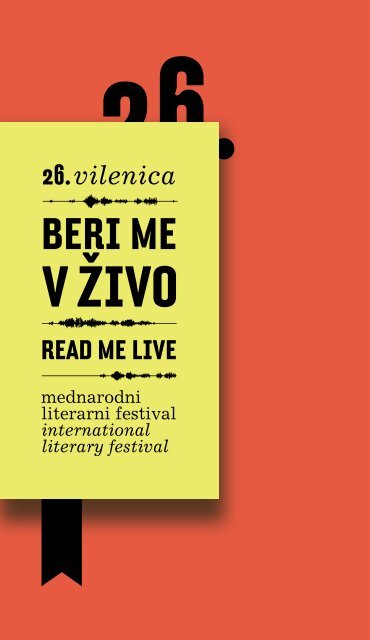This is an orange poster advertising an International Literary Festival. In the upper left center, there is a black number "26," partially covered by a yellow rectangle. The yellow rectangle features black text that reads "26 Valencia" at the top. Below that, there are different lines of text: "Bere mi visivo" (or possibly "Bury me gazebo"), followed by "Read Me Live," and "Madaroni Literary Festival." The text ends with "International Literary Festival." A black line, resembling the bottom of a ribbon, extends downward from the yellow rectangle. The poster seems to mix both Italian and English languages.